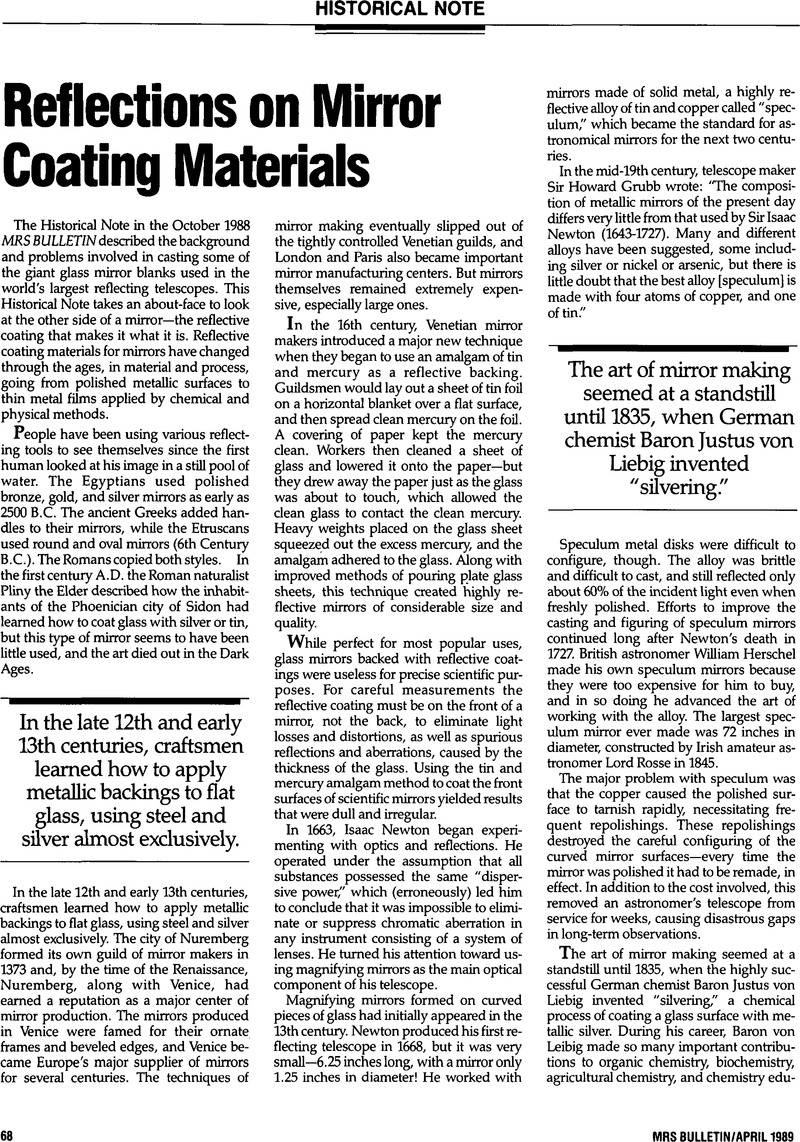This black-and-white image appears to be a reprint of a newspaper or magazine article, possibly from a book, given its format. The portrait-oriented image contains three columns of text on a plain white background without any borders. At the very top, the title "HISTORICAL NOTE" is displayed in all caps with a thick underline running beneath it, followed by a thinner underline stretching across the entire width of the image.

The headline for the article, "Reflections on Mirror Coating Materials," is left-justified and spans the two leftmost columns. Each column consists of several paragraphs, with the rightmost column extending almost to the top since it doesn't have the header above it. Notably, the beginnings of many paragraphs feature larger initial letters, commonly seen in printed articles.

Within the text, there are emphasized excerpts in larger font sizes. One such excerpt in the lower part of the left column states, "In the late 12th and early 13th centuries," followed by more text. Another prominent excerpt near the top of the rightmost column declares, "The art of mirror making seemed at a standstill," continuing with further lines of text.

At the bottom corners, there are additional details: the left corner mentions the page number "68," while the right corner indicates the publication, "MRS BULLETIN / APRIL 1989," all in caps.